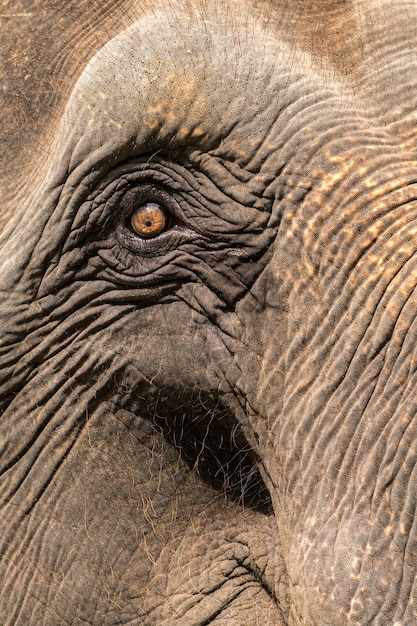The photograph is an extreme close-up of an elephant's face, capturing intricate details that emphasize its textured features. Dominating the image is the elephant's eye, which is round, yellowish-brown, and houses a dark black pupil at its center. Surrounding the eye are numerous creases and wrinkles, contributing to the deeply furrowed and aged appearance of the skin. The elephant's thick, gray skin shows subtle variations in color, with shades of white interspersed. A few fine white hairs can be seen towards the tip of the trunk, which extends down the right-hand side of the frame and out of view. The overall focus of the image is on the elephant's deeply wrinkled face and expressive eye, presenting a raw, intimate portrait of the majestic animal.